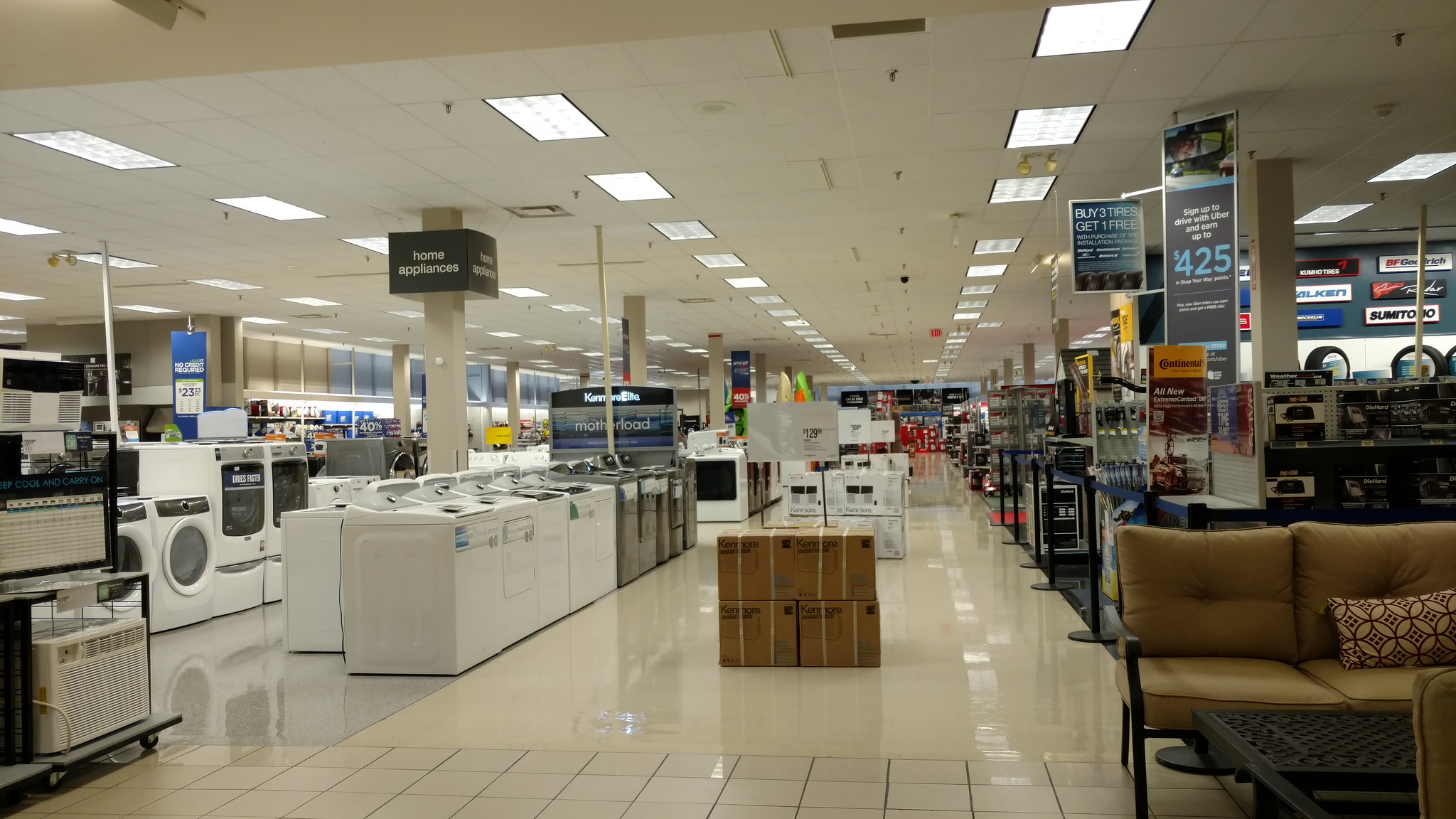This photograph captures the home appliance section of a large retail store, reminiscent of chains like Sears or Walmart. Prominently displayed, a sign reads "Home Appliances," marking rows of washers and dryers to the left, with labels indicating machines such as dryers. The middle aisle features various signs, including one advertising a promotion: "Buy three tires, get one free," and another with an unreadable text but showing a price of $425.

On the right side, the aisle transitions into a furniture display, with visible couches, assorted chairs, and throw pillows. Behind the furniture, there's a section displaying automotive parts, including tires and other car-related items. The store's floor is a shiny, reflective white linoleum, complemented by bright white fluorescent lights overhead, whose reflections are visible on the floor. The scene also includes additional water dispensers installed above the ceiling for fire safety. The overall ambiance is of a spacious and well-organized retail environment, with straight lines of home appliances and a blend of other merchandise extending from the front to the back of the image.